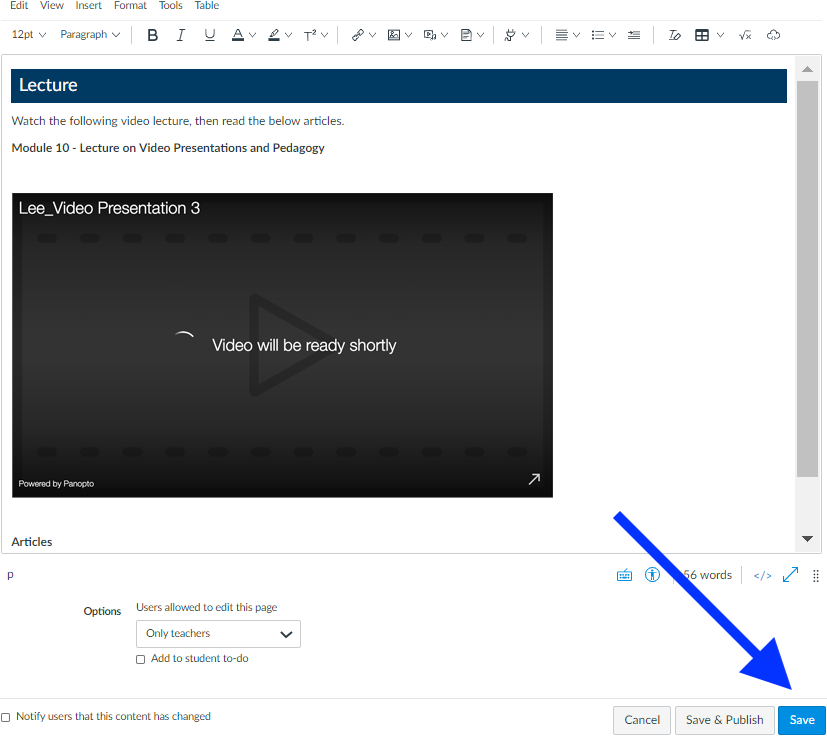This image appears to be a screenshot of an online presentation or learning management system interface with a clean, white background. In the top left corner, there are various menu tabs labeled "Edit," "View," "Insert," "Format," "Tools," and "Table." Below these tabs is a toolbar running horizontally across the entire image, displaying icons for text formatting, such as font size (12 pt.), paragraph settings, bold, italics, underline, text color, and additional formatting options.

Under this toolbar is a large rectangular box containing another smaller, dark blue rectangle with white text that reads "Lecture." To the right of this label, there's a vertical scroll arrow for navigating the page's content. Directly below the "Lecture" box, black text instructs users to "Watch the following video lecture, then read the below articles." The bolded heading beneath that reads "Module 10: Lecture on Video Presentations and Pedagogy."

Further down, there is a placeholder box for a video, labeled "Lee_video presentation 30," with the message "Video will be ready shortly" in its center. In the bottom left corner of the image, text states "Powered by," followed by a partially obscured word starting with "P-A-N-O." To the right of this text is a right-pointing arrow icon.

Below this section, there is a heading "Articles" followed by a drop-down box titled "Options." This box allows user permissions to be set, specifying that "Only teachers" are allowed to edit the page. It also includes two checkboxes: one labeled "Add to student to-do," and another "Notify users that this content has changed."

On the right-hand side, a blue, hand-drawn arrow points downward towards a blue "Save" button located at the bottom-right of the image. Adjacent to this button are additional options labeled "Cancel" and "Publish." The arrow is prominently pointing to the "Save" option.